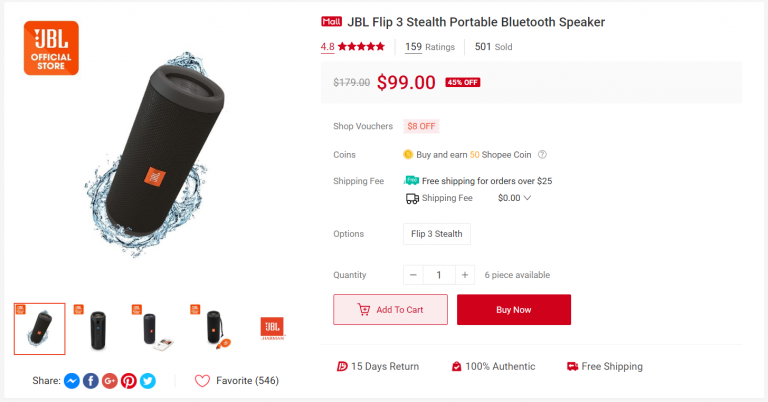**Detailed Product Description for JBL Flip 3 Stealth Portable Bluetooth Speaker**

Presenting a detailed glimpse into JBL's official store via a screenshot, showcasing the JBL Flip 3 Stealth Portable Bluetooth Speaker. This acclaimed speaker boasts an impressive rating of 4.8 stars, highlighting its popularity and quality among users. Currently available at a significant discount of 45% off, the price has been reduced from the original $179 to an attractive $99, making it a great deal for audiophiles.

Additionally, the store offers an $8 discount voucher, contributing further to potential savings. Purchases can also earn Shopee coins, adding value for frequent shoppers. With free shipping available for orders over $25, customers can enjoy their new speaker without incurring extra delivery charges.

The product page details various options, including the Flip 3 Stealth model, which may not be as flashy as some other versions but promises reliable performance. Customers can select a quantity of up to six pieces, with the current stock showing six available units.

For ease of purchase, there's a clear "Add to Cart" button in pink, and a prominent "Buy Now" button in red for quick transactions. Buyers can return the product within 15 days if unsatisfied, with assurances of 100% authenticity and the benefit of free shipping. 

On the right side of the page, shoppers can share the product on various social media platforms including Twitter, Facebook, Google+, and Pinterest. Additionally, there are four different viewing angles of the speaker at the bottom of the page, providing a comprehensive look at this sleek device.

This detailed breakdown captures the essence of the JBL Flip 3 Stealth Portable Bluetooth Speaker’s presentation and the exceptional deal currently available.